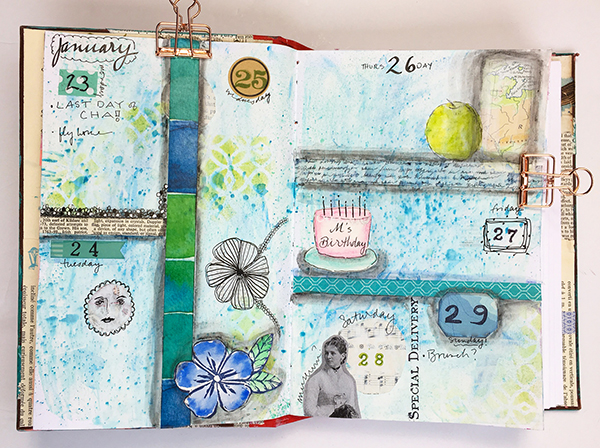This image depicts a meticulously crafted, colorful planner with a scrapbook-like feel, spread open to display the week starting January 23rd. The dominant hues are green, blue, and teal, with occasional splashes of yellow. Each day features unique hand-drawn decorations and notes. 

January 23rd is marked as the "last day" with the word "cha!" in lively handwriting. The 24th showcases a doodle of a sun or moon face, and January 25th features two elegant floral drawings: a detailed black-and-white flower with several petals and a vibrant five-petal blue flower with green leaves. 

On January 26th, a yellowish apple resembling a Granny Smith is drawn, accompanied by a map on the right side of the section. January 27th highlights a celebratory illustration of a pink birthday cake adorned with candles, labeled "M’s birthday." 

Saturday the 28th displays a Victorian woman in a choker, her head tilted left, in a striking black-and-white image. Finally, the 29th is marked with the casual query, "brunch?" in handwriting. The planner is laid against a white surface, possibly a table, and the layout of the days is inconsistent, adding to its quirky and personalized charm.